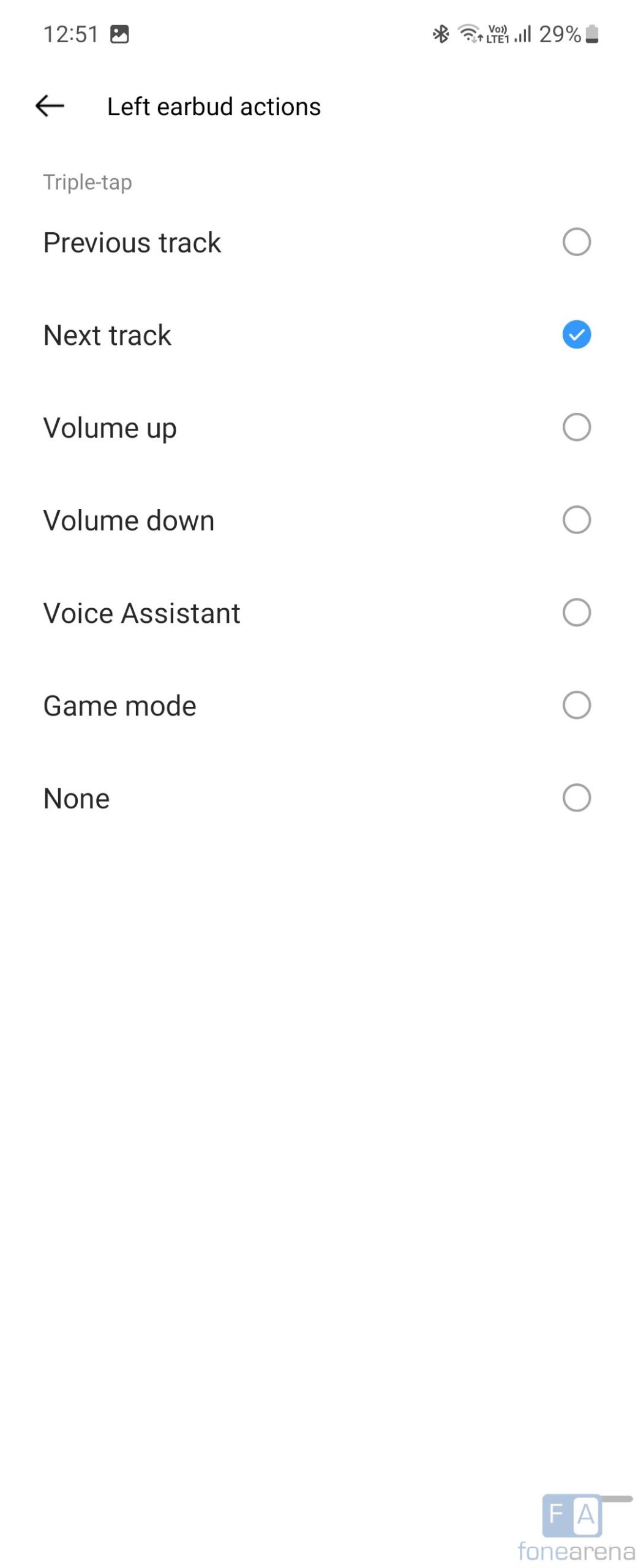This image is a detailed screenshot taken from a mobile phone, displaying an open menu against a white background with all text in black. At the top of the screenshot, the time is shown as 12:51 in the upper left corner. Adjacent to the time is an icon resembling a photo, which provides access to the phone's gallery. Moving to the right, several icons indicate the phone's status: the Bluetooth icon, the Wi-Fi icon showing three out of four bars, the mobile signal icon indicating full signal strength, and a battery icon displaying a charge of 29%.

Beneath these icons, the menu title "Left Earbud Actions" is prominently displayed in black font with a small arrow pointing to the left beside it. Below this title, in gray font, the instruction "Triple Dash Tap" is presented. Following this, there is a vertical list of options that appear in black text: "Previous Track," "Next Track," "Volume Up," "Volume Down," "Voice Assistant," "Game Mode," and "None."

To the right of each listed option, there are small empty black circles, which serve as selectable buttons. The selection for "Next Track" has been made, indicated by the circle turning blue with a white check mark in the center.